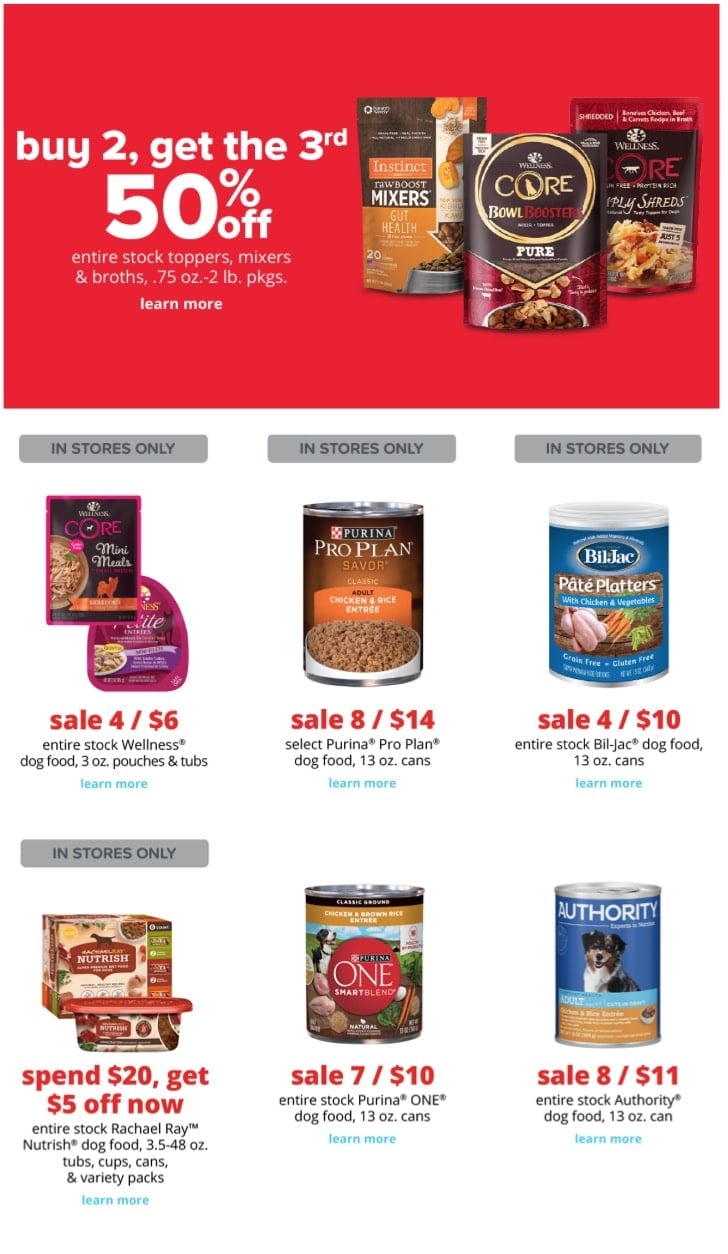Here is the revised, detailed caption for the image:

---

This is a screenshot of an e-commerce website showcasing a promotional offer and various dog food products. At the top of the image, a large red rectangle with bold white text announces a special deal: "Buy two, get the third 50% off entire stock of toppers, mixers, and broths, 0.75 ounce to 2-pound packages, and more."

Below the promotional banner, there are three pictures of different bags of dog food. Underneath these images, a white rectangle features a layout of six items for sale, arranged in two rows of three. Each item has a descriptive label and sale information:

**First Row:**
1. On the far left, there is a label "In-store only" above an image of a bottle. The text indicates a sale: "4 for $6 on the entire stock of Wellness dog food 3-ounce pouches and tubs."
2. In the middle, a can of dog food labeled "In-store only" is showcased. The sale reads: "8 for $14 on select Purina Pro Plan dog food 13-ounce cans."
3. On the right, another can is featured with the label "Sale 4 for $10 on the entire stock of Bil-Jac dog food 13-ounce cans."

**Second Row:**
1. On the left, another "In-store only" label highlights a promotion: "Spend $20, get $5 off on the entire stock of Rachael Ray Nutrish dog food."

The combination of deals and product images gives a clear view of the ongoing sales and promotions on various dog food items.